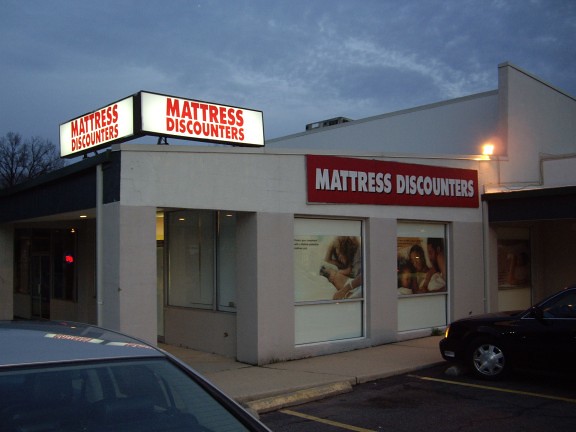This photograph captures the corner of a commercial building constructed from white concrete. The base of the building is composed of a slightly darker concrete, providing a subtle contrast. Above two windows on the front facade, a prominent red sign with white letters proudly announces "Mattress Discounters." The windows themselves are adorned with posters: one displays a family, another features a couple sitting together, and the third shows a woman holding either a baby or a dog. At the top corner of the building, a white sign reiterates "Mattress Discounters" along each edge, ensuring visibility from multiple angles. In the foreground, a silver car is parked to the left, while a black car occupies the right side of the image.